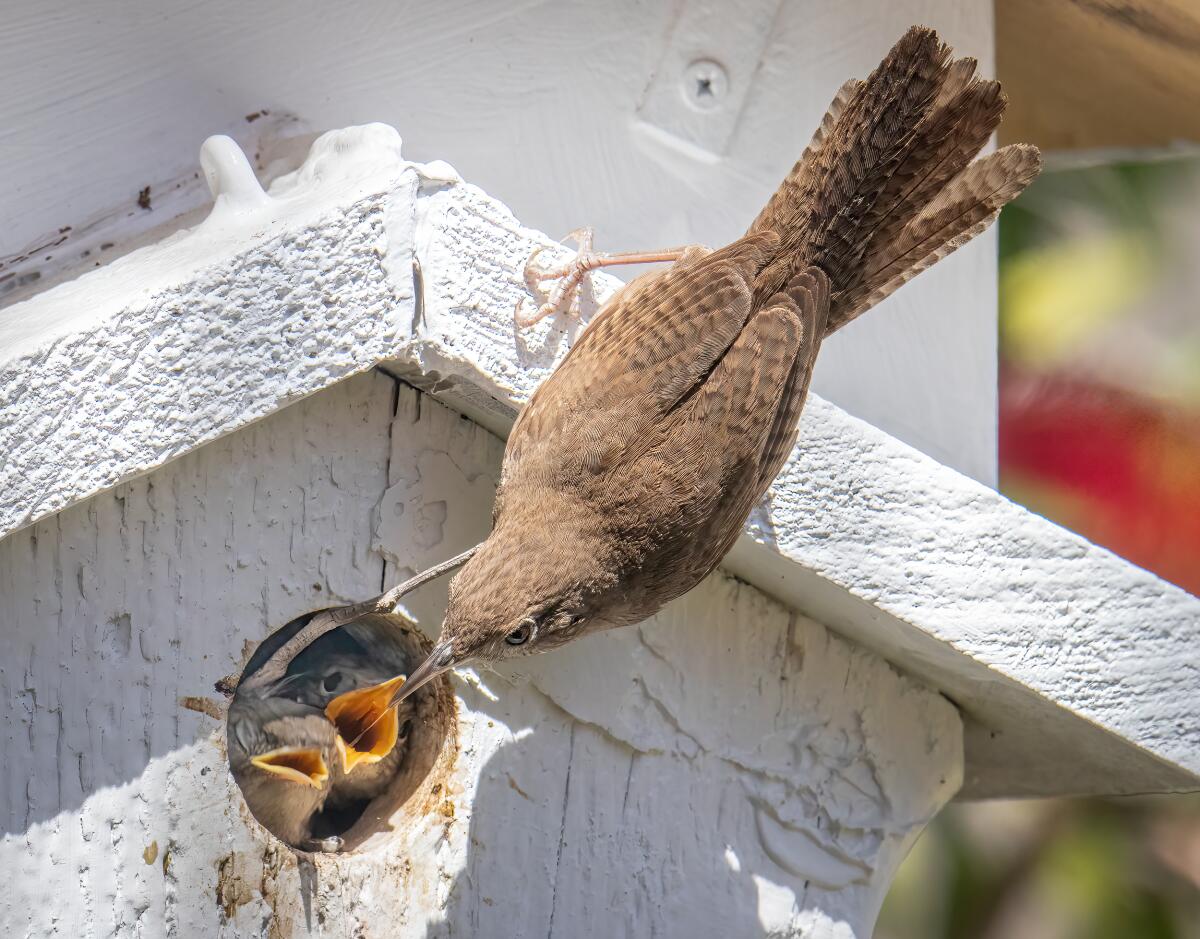In this captivating image, a mother bird, likely a sparrow with light brownish-gray plumage and detailed darker brown striping on its wings and tail, is seen feeding her two baby birds. The mother bird has a long, thin beak and is perched almost upside down on the white, triangular roof of a handmade, white-painted birdhouse. Her beak is reaching into a small, precisely drilled hole in the birdhouse from which the two baby birds eagerly stretch their fuzzy, dark gray bodies and open, vibrant yellow-orange beaks. Surrounding the birdhouse is a wooden area painted white, displaying some signs of wear. A painted metal bar, fixed with a screw, suggests that this birdhouse is securely attached, likely to a house or a tree. The background includes subtle hints of greenery and a blurry, possibly red flower, adding a touch of natural color to the scene. The close-up focus emphasizes the tender moment of the mother feeding her chicks, their outstretched beaks waiting for the next morsel.